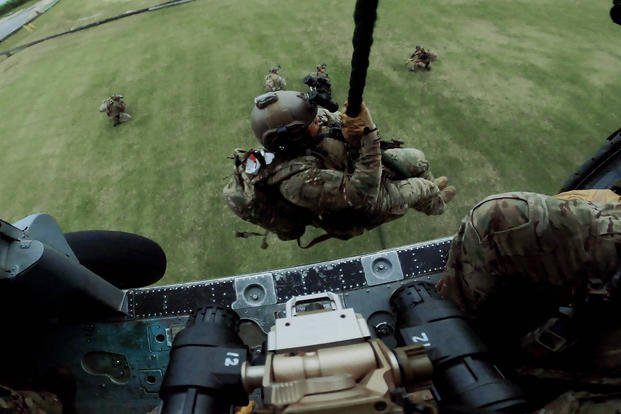In this horizontally-oriented, realistic photograph taken from about 100 feet in the air, likely from inside a military helicopter, we see a Marine dangling from a black rope, preparing to rappel down to the light green grassy ground below. The Marine, dressed in an olive and beige uniform with an olive helmet, appears to be either climbing down or up the rope. Surrounding the dangling Marine are other personnel on the ground and potentially a leg of another camouflaged soldier next to the photographer, whose perspective is from the edge of a metal platform, possibly indicated by the presence of a wheel suggesting a helicopter. The ground below features green grass and possibly bushes, camouflaged soldiers, or both, and it appears to be a military training exercise. There is no text in the image, except for the number "12" in white font on some equipment inside the helicopter.